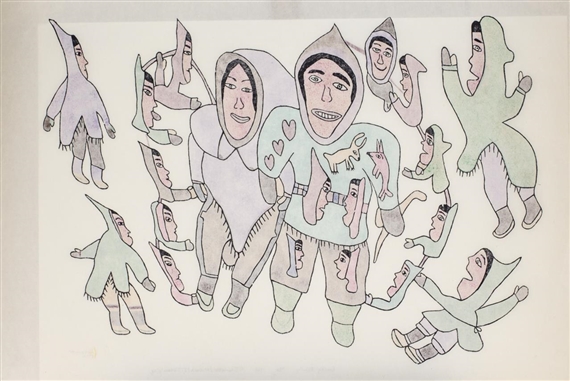This detailed piece of surrealist, impressionist art features a group of cartoonish, miniature people predominantly painted in neutral tones—black, white, gray—with very pale shades of light blue and pink, almost blending into the white background. Central to the image is a woman on the left and a man on the right, both with short black hair and dressed distinctively. The woman wears a purple top and brown trousers, accompanied by a headscarf and small boots. The man, her mate, is adorned in a teal top with brown trousers and green shoes, embellished with intricate patterns including hearts, faces, and deer. Surrounding this central couple are numerous smaller versions of themselves, giving an impression of either their children or an echo of their own images. These miniature figures, dressed similarly in pointed hood-like garments, appear joyous, reaching towards the central figures with smiles and raised hands. Their detailed expressions and attire, similar to the central duo's, create a whimsical and dream-like atmosphere, reminiscent of something out of a fever dream or a Picasso-inspired fantasy.